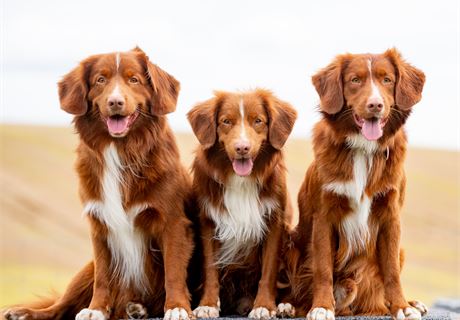This is a vibrant vertical rectangular image taken outdoors during the daytime, likely at a beach. The upper half of the image features a light blue expanse that could be either the sky or ocean water, complemented by a light brown sandy background. At the forefront, three dogs are positioned in a horizontal row, facing the camera with their mouths open, tongues hanging out, and eyes fixated ahead. These dogs, which might be related due to their strikingly similar appearances, resemble breeds like Irish Setters or Golden Retrievers but with slight differences in their fur.

The dogs are primarily reddish-brown with long, fluffy ears and tails. They each have distinct white markings: a stripe down the middle of their foreheads and noses, white fur on their chests, and white-tipped paws. The two larger dogs flank a smaller one in the center, giving a sense of familial hierarchy. Their identical reddish-brown hues and identical white accents make them appear almost identical despite the differences in their sizes. The image captures a moment of lively attention from the trio, set against the serene backdrop of what is presumably a beach.